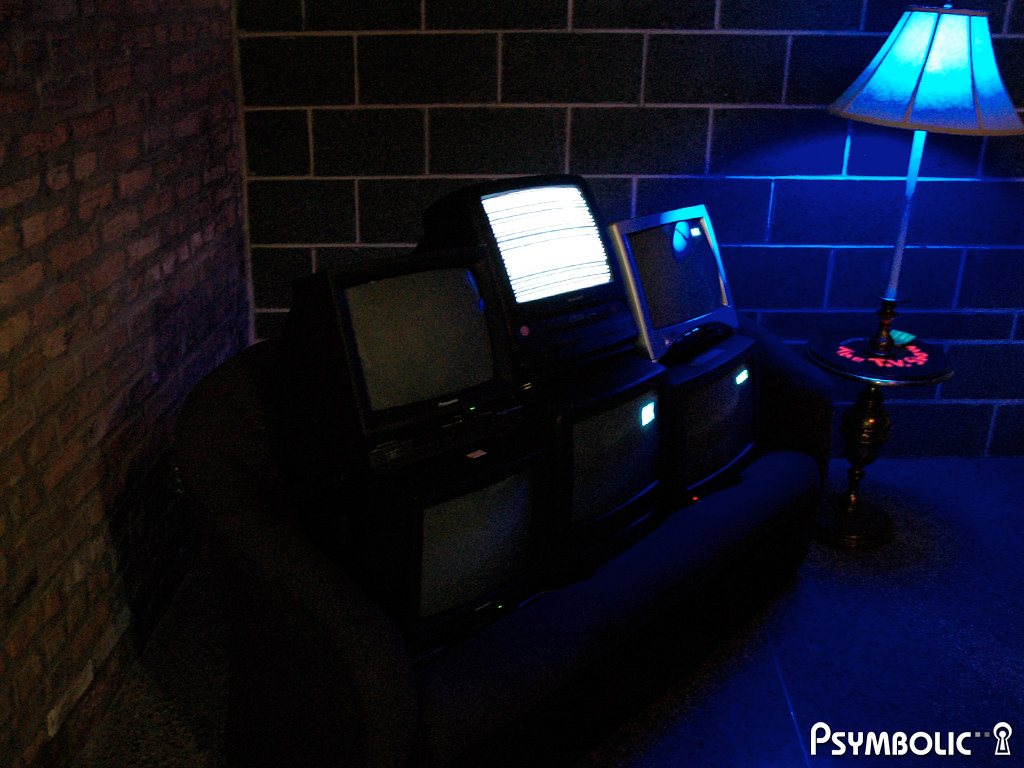In this dimly lit room, giving off a chill ambiance, we observe a setup where a two-seater black couch is positioned facing around four o'clock. Resting on the couch is a grid of six old-school, square, mid-90s style TV monitors, each approximately 19 to 22 inches. The monitors are arranged in two rows of three. Out of these, only the middle monitor on the top row is on, displaying a glitchy image, while the rest have their screens off, showing only black bezels. To the side of the couch stands a side table with a tall lamp that emanates a blue glow, adding to the room's dark and eerie atmosphere. The room's left wall features worn red bricks, and the far wall, barely distinguished due to the dim lighting, showcases horizontal rectangular tiles with whitish grout. A watermark or credit labeled "Symbolic" along with an old-fashioned keyhole logo is prominently displayed at the bottom right corner of the image.